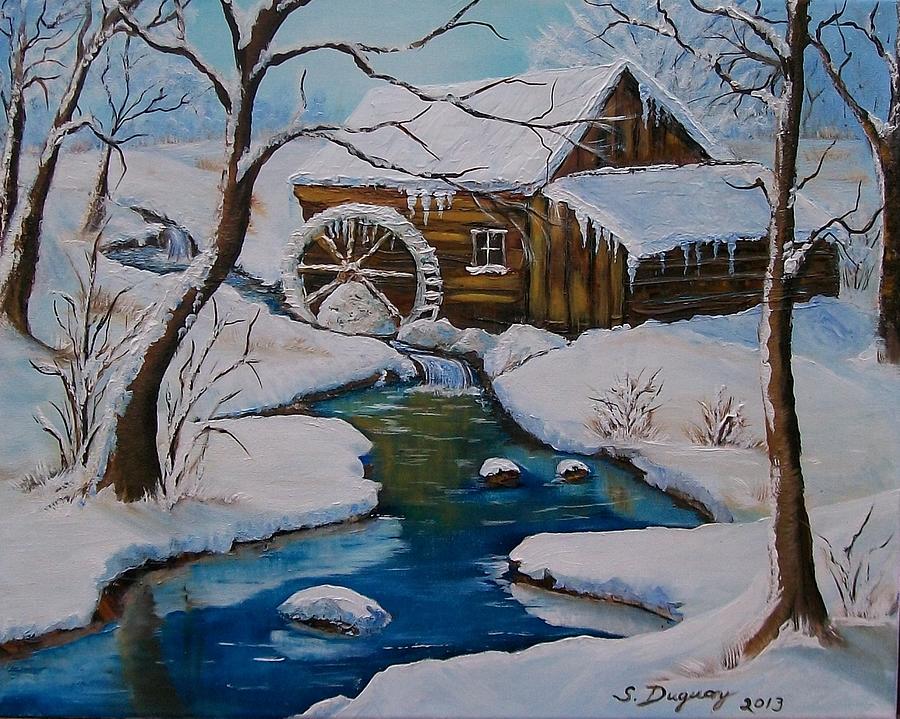This detailed painting captures a serene winter scene featuring a rustic brown log cabin, reminiscent of an early American gristmill, nestled by a flowing stream. The cabin, positioned in the upper center of the painting, showcases a distinct V-peaked roof and has one visible four-pane window. Both the rooftop and the adjacent lean-to shed are thickly blanketed with snow, dripping icicles adding to the wintry atmosphere. A prominent feature of the cabin is the large, snow-covered paddle wheel, partly submerged in the dark, intense ultramarine and cobalt blue water of the stream. The stream, with snow-covered rocks and small cascading waterfalls, winds through the snowy landscape.

Flanking the stream are bare trees, starkly devoid of leaves but heavily laden with snow. These trees frame the cabin—four to the left, two to the right—and extend into the background, creating a dense thicket. The shoreline is dotted with patches of brown, possibly dead weeds, poking through the pristine snow. Above, a bright, clear blue sky suggests the calm following a snowstorm, enhancing the tranquil beauty of the scene. The painting is signed in black script at the bottom right corner, reading "S.DUGUAY 2013," cementing its authenticity and the year of its creation.